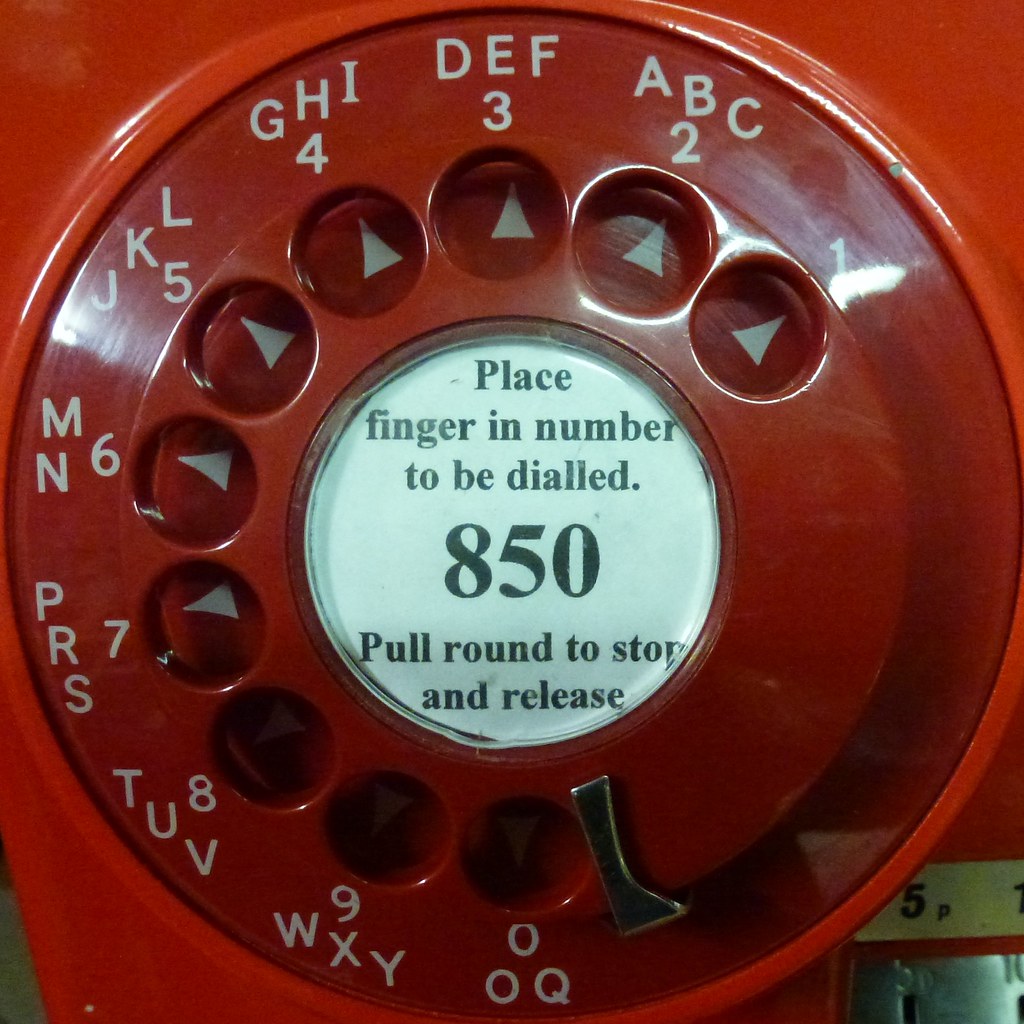This is a detailed close-up color photograph of an antique red rotary phone. The focus is on the circular rotary dial, which is predominantly red with white text and numbers. Within the center of the rotary dial, there is a clear window displaying a white piece of paper with black instructions that read: "place finger in number to be dialed 850, pull around to stop and release," detailing the dialing process. The text "Dialed" is notably spelled as "D-I-A-L-L-E-D." The upper half of the dial features various labels indicating the corresponding letters and numbers, such as "DEF 3" at the 12 o'clock position, "ABC 2" to the right, and others continuing around the dial in a clockwise manner. This vintage phone, made of strikingly red plastic, appears well-preserved and might be considered a museum piece, reflecting a bygone era when such dialing mechanisms were commonplace.